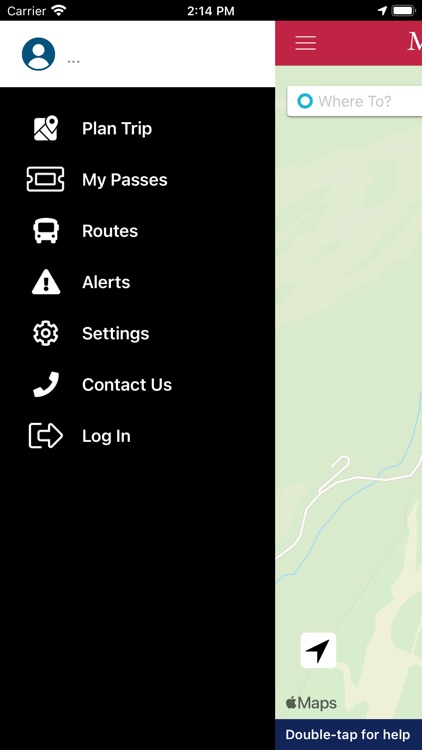The screenshot showcases a website displayed on an iPhone, with the time prominently shown as 2:14 PM and the phone indicating a full battery. The carrier information is visible as "Carrier," indicating the phone's service provider. The main visual element is a generic blue profile icon of a person on a white background. 

To the right of the profile icon is a partly visible red bar containing three horizontal lines and an "M" in white. Below, a vertical green section features the phrase "Where to?" accompanied by a blue circle and an undetailed map. The map is depicted with shades of green, a blue line, a white line, and a general land outline, labeled "Apple Maps." A prompt at the bottom encourages users to "double tap for help."

On the left side, a black sidebar lists various options in white text, each with corresponding icons:
- Plan Trip
- My Passes
- Routes
- Alerts
- Settings
- Contact Us
- Log In

The website appears incomplete on the iPhone screen, notably cutting off half of the map and the red bar on the right side.